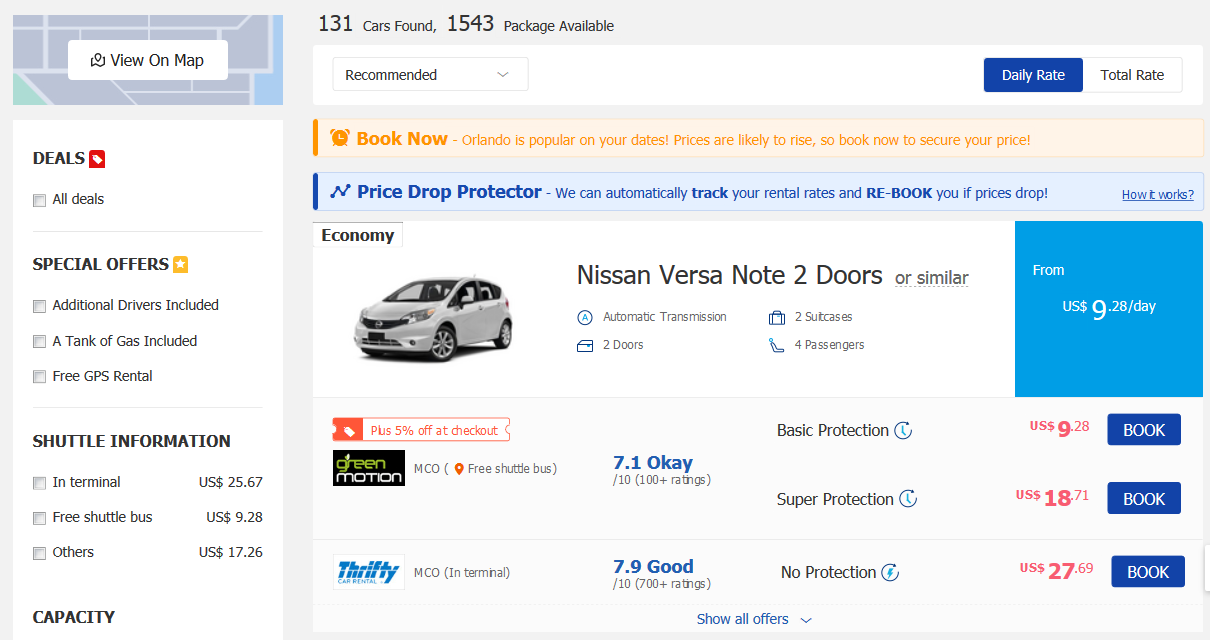The image appears to be a detailed screenshot of a car rental booking section on a website or app, displaying various features and options available for users. 

On the left side of the image, there's a vertical sidebar. At the very top of the sidebar, a map is partially visible within a box, containing a white button labeled "View on Map." Beneath this map box, there is a section with categories like "Deals" and a checkbox labeled "All Deals." Following this, there is a "Special Offers" category with three different options, each accompanied by checkboxes.

Further down, another category titled "Shuttle Information" appears with three subsequent subcategories. Toward the bottom of the sidebar, there is a "Capacity" category.

The main content on the right-hand side features prominent booking and pricing details. A white bar at the top of this section reads "Recommended Daily Rate" in a blue box, and "Total Rate" in a white box. Below this, an orange box spans across the screen with the text "Book Now" and additional details. Just underneath, a blue bar labeled "Price Drop Protected" extends across with accompanying text.

Following this, there's a white box presenting detailed information about a car. It includes a photograph of a gray Nissan Versa with a description reading "Two doors," along with specifics about the car. To the right of the car image, a blue box displays the rental price starting from "US $9.28 a day" in white text. 

Beneath the Nissan Versa details, two additional car options are listed. These entries include a small icon on the left, descriptive text to the right of the icon, user ratings, protection plan information, pricing, and a booking button on the right side of each entry.